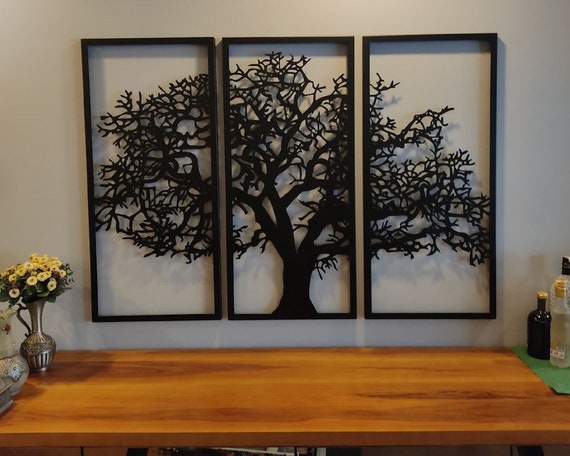The image displays a serene and meticulously arranged setting, featuring a light brown wooden table partially visible at the bottom. On the left side of the table, there are two flower vases, one silver and one brown, both with yellow flowers inside. The right side of the table is adorned with three drink bottles, including a black bottle and a clear one. 

Above the table hangs a striking three-sectioned artwork, each black-framed vertical rectangle forming a continuous image of a leafless tree. The central panel showcases the thick trunk and spreading branches, while the side panels feature the extended branches, all in black against a white background. The harmonious use of colors—black, white, yellow, green, and brown—creates a crisp, balanced composition without any text.